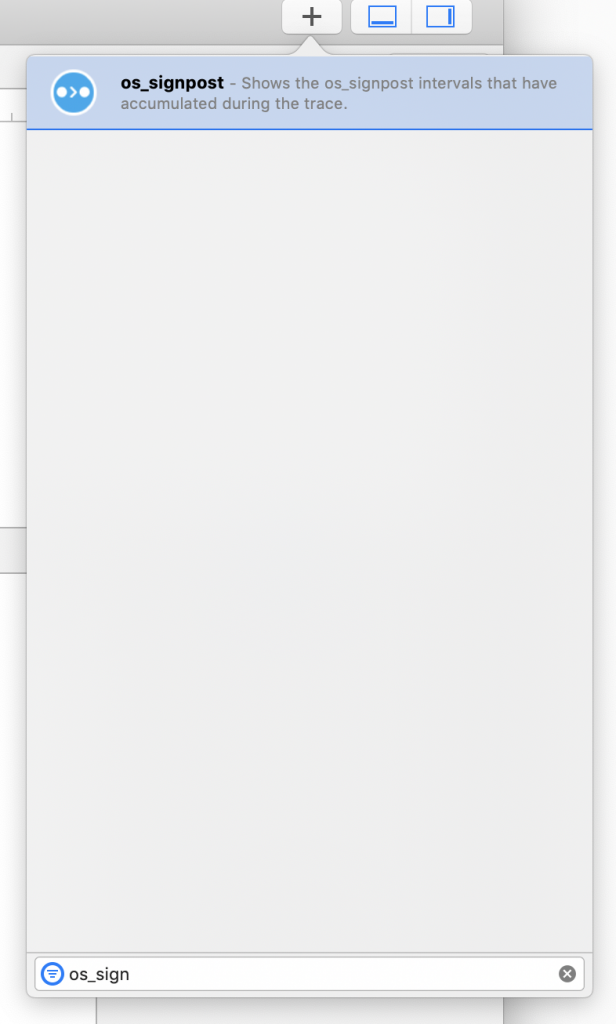The image displays a complex interface focused on illustrating the accumulation of OS sine post intervals during a trace. Central to the interface is a prominently grey area, which is flanked at the bottom by a blue circle containing a white cross symbol. Surrounding this central area, there is an array of contextual information and symbols, including several windows showcasing a variety of graphical indicators. These include squares, vertical lines, and arrows, all seemingly part of a structured layout designed to convey detailed timing and interval data. The overall color scheme features predominantly white edges, interspersed with grey tones and blue highlights, giving the interface a clinical and data-focused appearance.